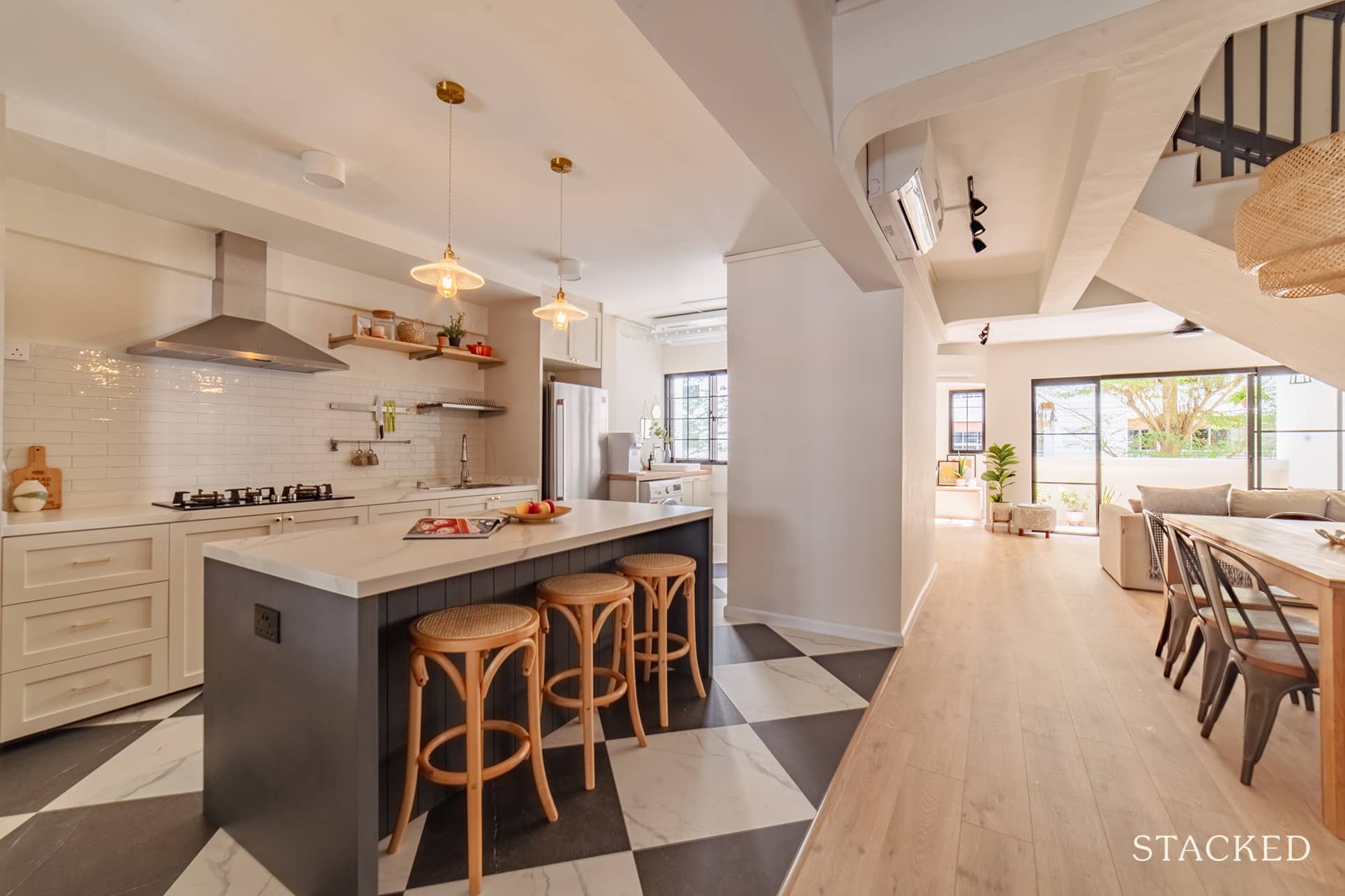This detailed photograph captures the interior of a house, focusing on the spacious kitchen and dining room areas. The kitchen, situated on the left side, features a black-painted wooden counter with a white marble countertop. Three bar stools are neatly tucked beneath the counter, which also houses a six-burner stove. A sleek convection air vent is mounted above the stove, paired with a sink in the far left corner, and a stainless steel refrigerator against the wall. Hanging lights from the ceiling cast a warm, yellow glow over the entire room, enhancing its inviting atmosphere. The kitchen floor is adorned with white and black tiles, contrasting with the warm brown wooden floor that extends throughout the rest of the house. On the right side of the room, there is a wooden dining table accompanied by six chairs with industrial-style legs. The bright, white-painted walls and the well-placed windows and door on the front wall add to the room’s airy and open feel. In the top right corner, a glimpse of the stair area is visible. The bottom right corner of the image features the word "stacked" in white lettering.